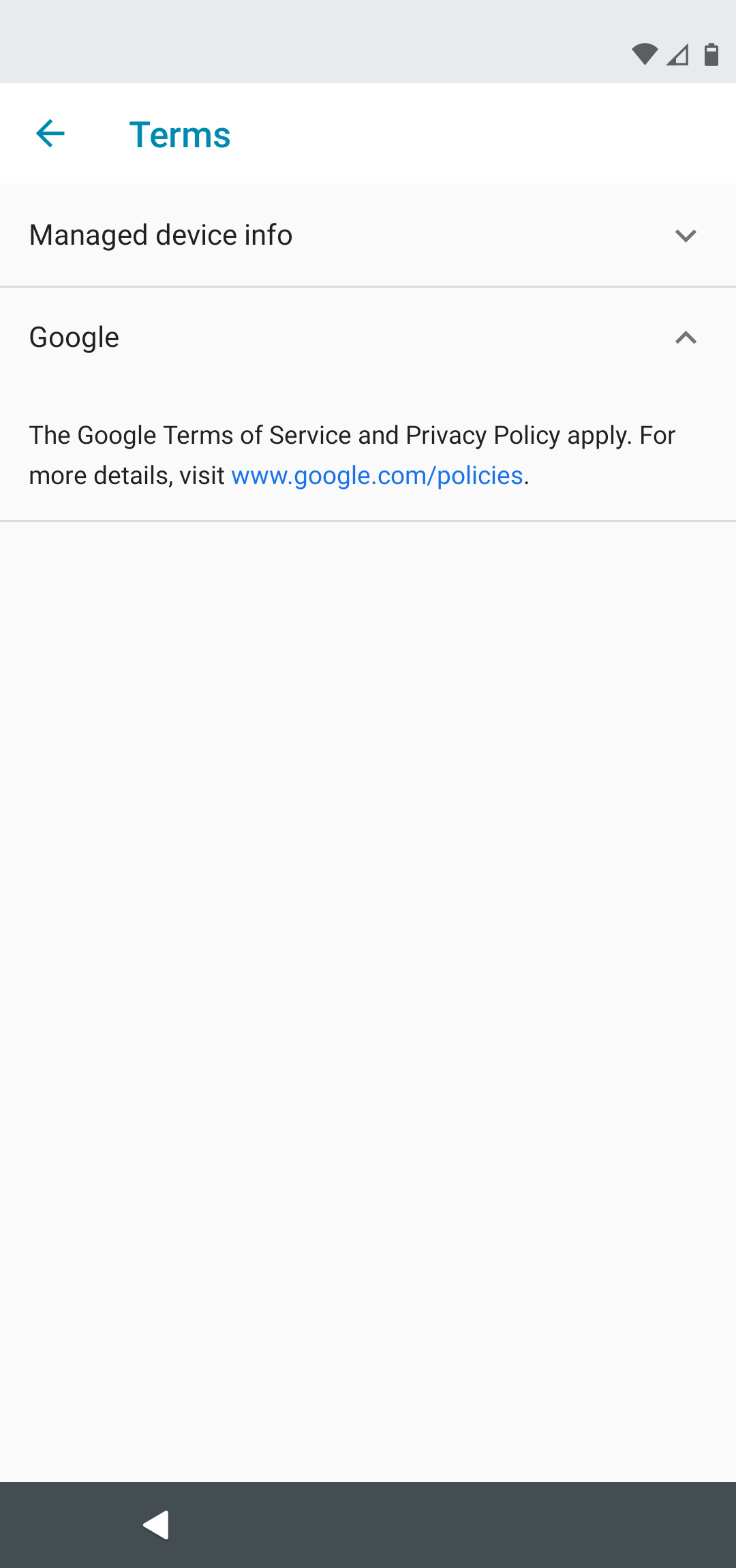The image appears to be a screenshot taken from a phone, characterized by its rectangular shape and various interface elements. At the top, there is a faded horizontal rectangle containing three symbols on the right: a pie chart section, a triangle with a shaded lower corner, and a battery icon that is approximately three-quarters full. 

Below this, the word "Terms" appears in a light aqua blue color with an arrow pointing left next to it. The background in this section is light gray. Further below, it reads "Manage Device Info" followed by a small "V" and a light horizontal gray line underneath. 

Continuing downward, the text "Google" is displayed with an inverted "V" to its right. Accompanying this are the words, "The Google Terms of Service and Privacy Policy Apply. For more details, visit www.google.com/policies."

At the bottom of the image, there is another rectangular area filled with a solid gray color. Within this area, there is a white triangle pointing to the left.